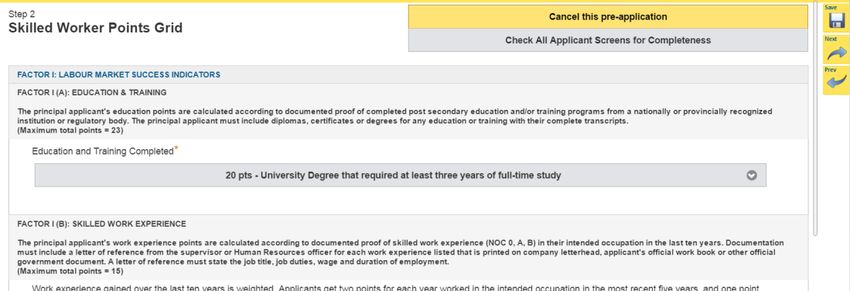This image contains a detailed overview of the criteria and documentation required for assessing a principal applicant's eligibility for skilled worker programs. The primary elements highlighted are: 

**Digital Text and Skilled Worker Points Grid:** The image features a grid that allocates points based on various labor market success indicators, focusing on education and training.

**Education and Training Requirements:** Points for the principal applicant's education are calculated according to documented proof of completed post-secondary education or training programs from nationally or provincially recognized institutions or regulatory bodies. The application must include diplomas, certificates, or degrees, along with complete transcripts. The maximum achievable total points for education is 23.

**Skilled Work Experience:** Points for the applicant's work experience are calculated based on documented proof of skilled work in the intended occupation within the last ten years. Required documentation includes reference letters from supervisors or human resources officers for each listed work experience, printed on company letterhead. These letters must detail the job title, job duties, wage, and duration of employment. Additional official documents such as the applicant's workbook or other government documents may also be required.

The comprehensive breakdown ensures clarity on the point allocation process for education and skilled work experience, emphasizing the need for precise documentation to support the applicant’s credentials.